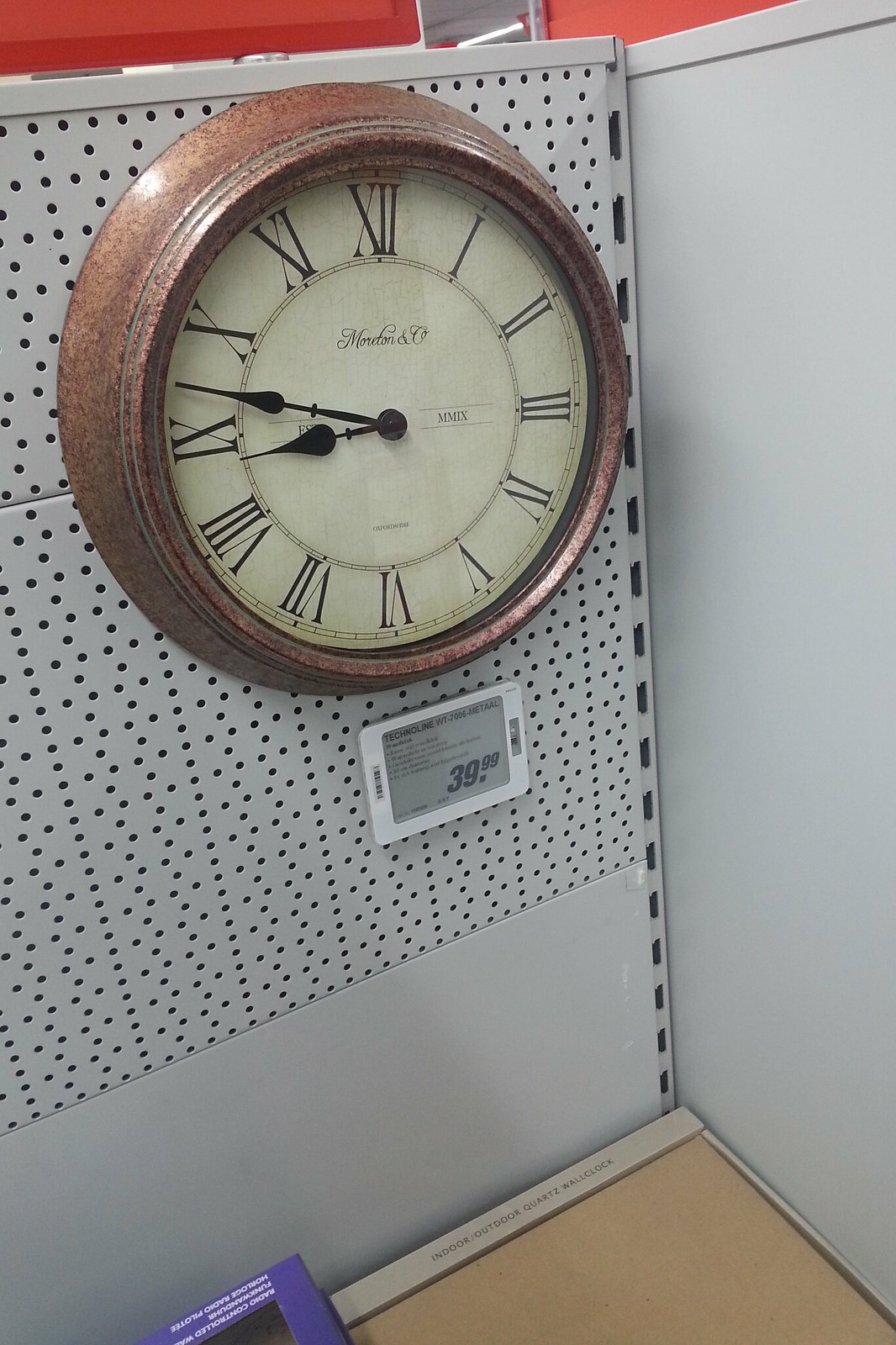This photograph captures a detailed store display featuring an antique-style wall clock mounted on a perforated metal shelf typically used in retail environments due to its versatile design with multiple holes for hanging items. The clock, which is a thick bronze piece with an ivory-colored face, displays large Roman numerals and black hands with spade-like tips, indicating the time as 8:47. A name in cursive is inscribed in the center of the clock, possibly reading "Morton and Company," although it is not entirely clear. Below the clock, a white tag holder contains a dark gray price tag stating the clock is priced at $39.99. The back of the clock is whiter compared to its face. Surrounding the display are additional shelves and products, including one in a blue box, under a well-lit area. The metal shelf, with its numerous holes, efficiently supports the clock for easy viewing and purchase.